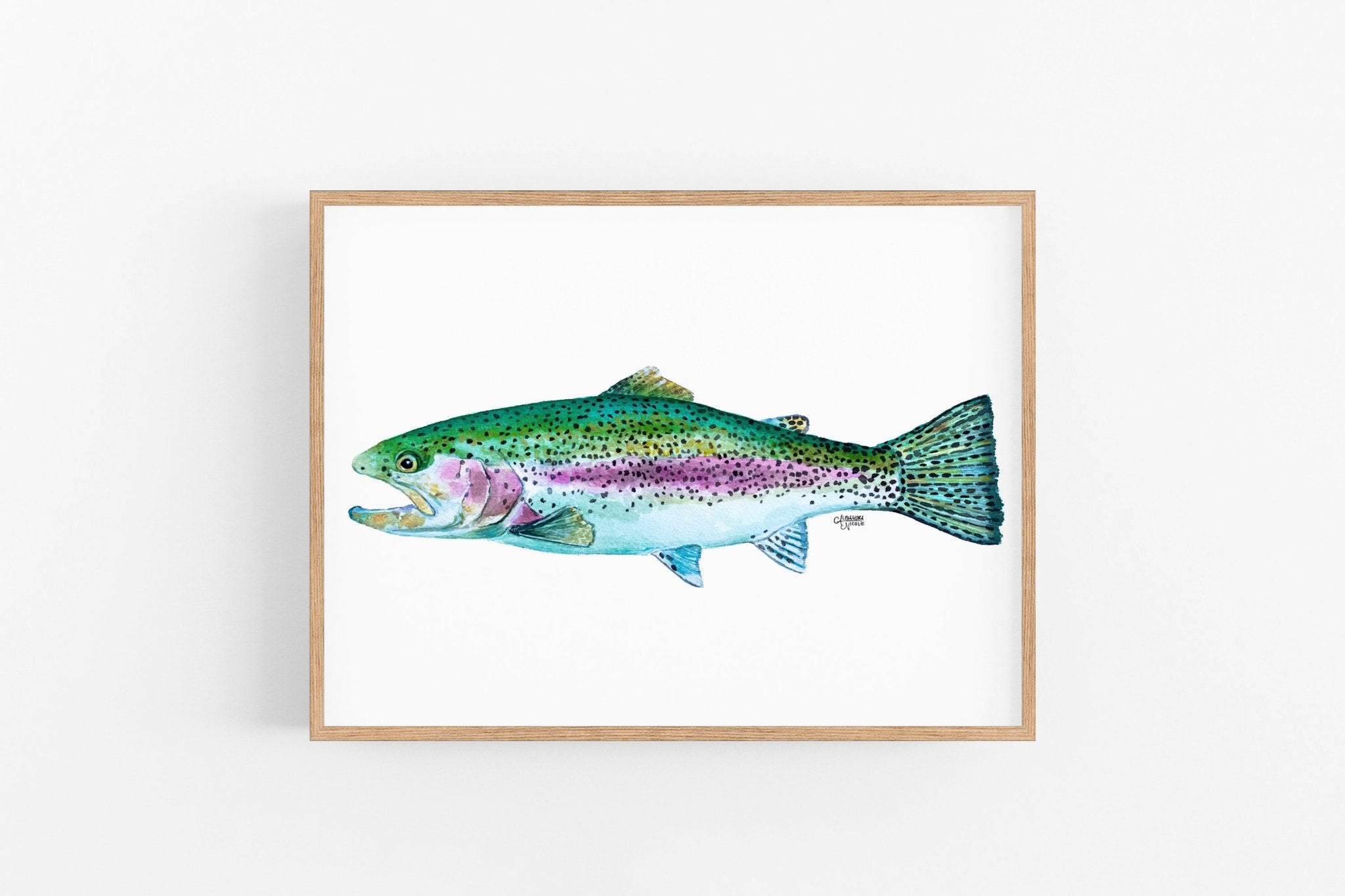The image showcases an artwork centered on a plain white background. The piece, resembling a watercolor painting, is encased in a thin light brown wooden frame and displays a colorful depiction of a rainbow trout. The fish is oriented with its head on the left and its tail on the right, almost spanning the entire width of the square-shaped frame, with minimal space on either side. The rainbow trout exhibits a myriad of colors: its gills and a central stripe down its body are purple, the belly and bottom of the mouth are light teal and white, and the top is a blend of dark green, teal, and touches of yellow or gold. The tail fin combines teal green and yellow hues, while the bottom fins are bluish white, and the top fins mix dark green, light green, and yellow. Notably, the fish's body is covered in hundreds of tiny black polka dots, particularly dense on the top half and more sparsely distributed on the tail fin, bottom fins, and top right fin. An initial, though barely legible due to its small size, is located near the tail. The shadow of the frame is faintly visible on the left side of the image, adding a subtle depth to the otherwise minimalist backdrop.